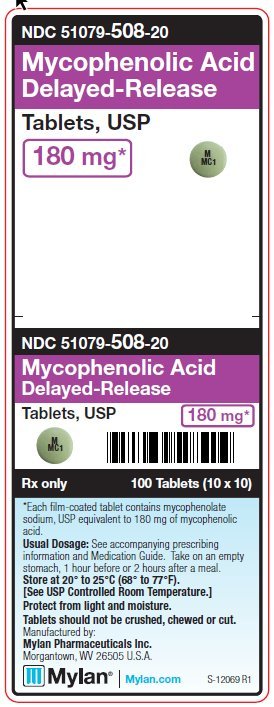At the top of the image, a long black bar features the text "NDC 51079-508-20" in all capital letters. Below this, set against a purple background, is the text "MYCOPHENOLIC ACID DELAYED-RELEASE TABLETS USP" with "tablets USP" set within a white square. Beneath this, within a purple rectangle, it reads "180 milligrams *". A small green pill is depicted to the right of this text.

Further down, within another white box, the text reiterates "tablets USP" alongside another image of the green pill, which bears a capital "M" inscription. Adjacent to this is a barcode and the designation "RX" indicating the medication is prescription-only. It states "100 tablets (10X10)" in parentheses.

At the bottom, the medication's dosage instructions are provided in a blue box, advising that tablets should neither be crushed, chewed, nor cut. Additional information is given about the manufacturer: "Manufactured by Mylan Pharmaceuticals, Incorporated." Finally, the image concludes with "Mylan.com" in blue at the very bottom.